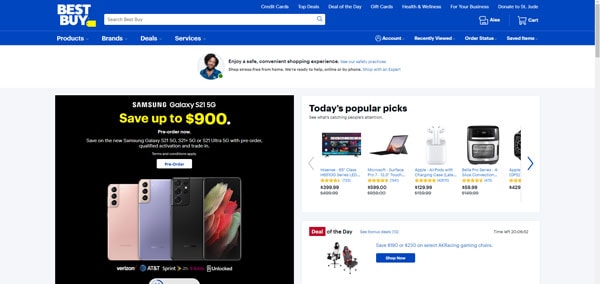The image depicts a section of the Best Buy website advertising Samsung Galaxy S21 5G phones. The topmost section features a blue banner with the "Best Buy" logo prominently displayed in white letters. Adjacent to the logo, there is a search bar followed by clickable menu options in light blue text, which are not clearly legible. Toward the right side of the banner is a cart icon.

Just below this banner, on the left, the website lists categories such as "Products," "Brands," "Deals," and "Services" in white text. Additional menu options extend to the right but are too small to read clearly. The main body of the webpage has a white background. It features an image of a woman with some accompanying text that is not legible.

To the left, a large black square prominently displays an offer for the Samsung Galaxy S21 5G, highlighting a savings of up to $900 in bold yellow text. Below this, there are additional details and a button, though the text is not readable. The product images include three phone colors: pink, light purple (or lilac), and black, plus a phone displaying its front screen with an image. Beneath these phones, there are logos for Verizon, AT&T, Sprint, T-Mobile, and an unreadable fifth logo.

On the right side of the page, a section titled "Today's Popular Picks" showcases images of a TV, a computer, an air purifier, and an air fryer. Beneath this, another section seems to feature images of office chairs, though the accompanying text is not legible.